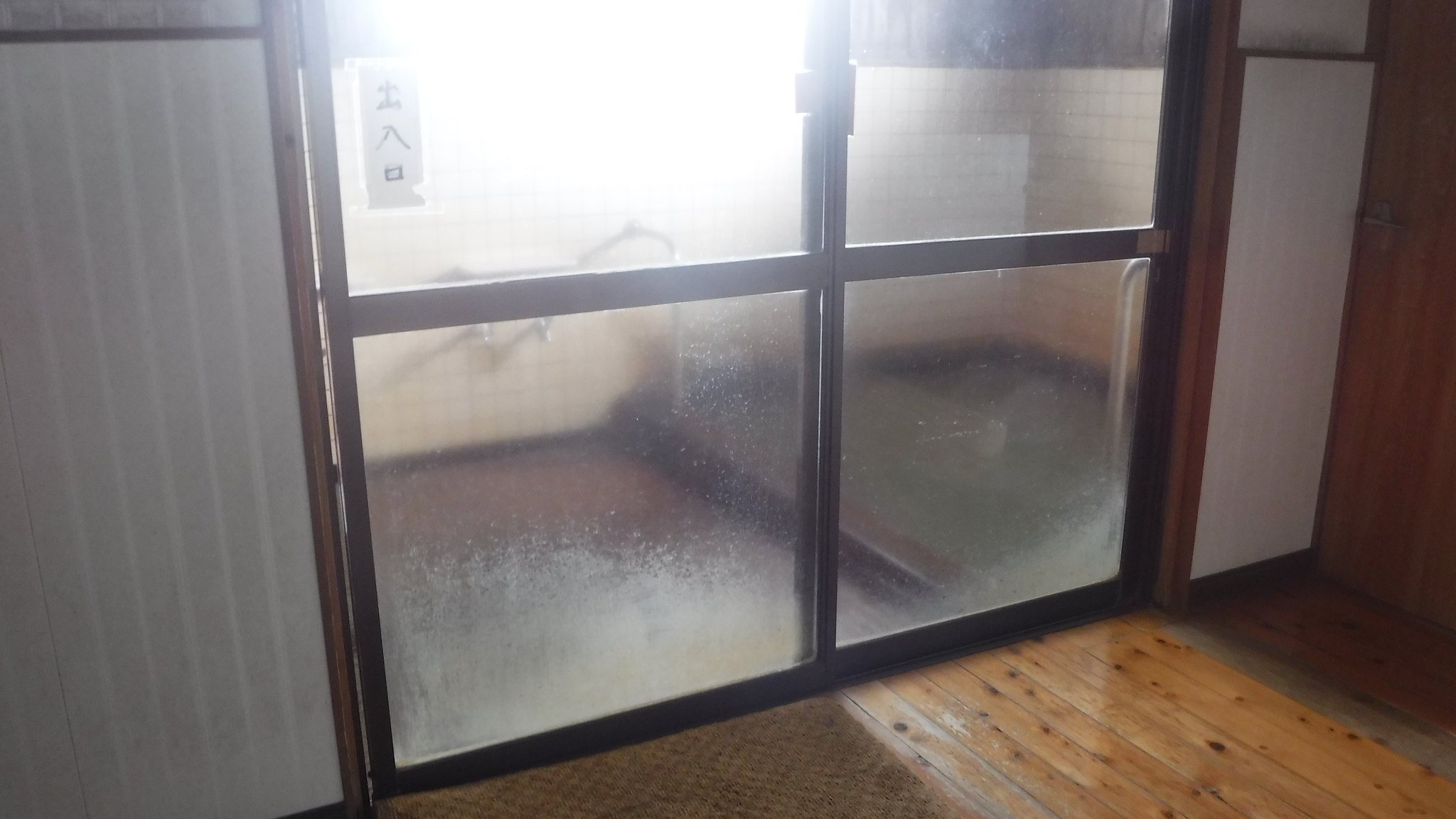The photograph captures the interior of a presumably Japanese home, divided by sliding glass doors. The central focus is a brown doorway with frosted and smudged glass featuring a light coffee-colored smear. Through the glass, a silver metal handlebar is visible. The doors appear to divide a main room from what looks like a sauna or a small shower room.

In the background, a white piece of paper with vertically arranged Japanese characters - thought to say "runko" which suggests an entrance in Chinese - is affixed to the left side of the glass. Sunlight streams through the scene, highlighting the contrasting textures and colors: a gray tile floor, walls that shift from white-striped on gray outside the sauna to a combination of yellow, brown, and black tiles inside.

The room beyond the doorway is unfurnished except for what looks like a bed or platform with a green cover and a square-shaped sauna, suggesting it functions as a relaxation space. The walls are white tile on the top with darker segments and a significant light source reflects off various surfaces, enhancing visibility. Overall, the image presents a tranquil environment typical of Japanese interior design, blending traditional elements with functional modern spaces.